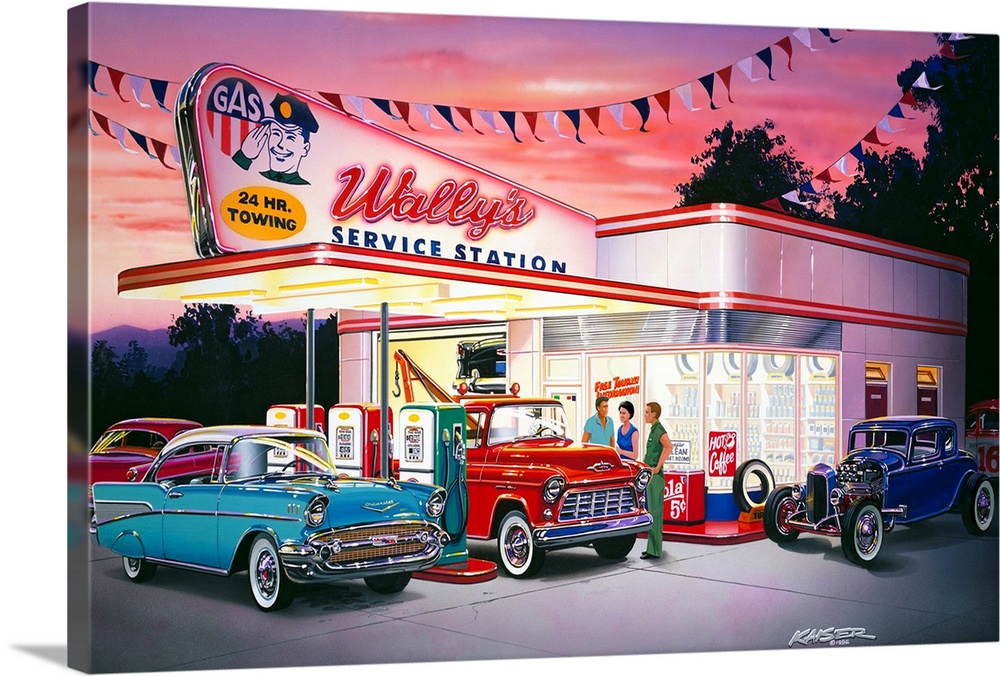In this vibrant and nostalgic scene set at sunset, we see an artist's detailed interpretation of Wally's Service Station, capturing the essence of the 1940s and 1950s. The sky is ablaze with hues of purple and orange, tinged with pink clouds, casting a warm glow over the scene. Two strings of flag banners, red, white, and black, stretch across the top, adding to the vintage charm.

The service station itself is a white structure with large front windows, punctuated by red stripes near the top and bottom. A roof overhang shelters the green and red gas pumps, and prominently displayed above is a sign reading "Wally's Service Station." This sign features a yellow circle with "24-hour towing" and a saluting man in a police hat. 

On the left side of the station, a garage bay is visible. In front of the gas pumps stands a classic 1950s blue Chevrolet with a white top, black wheels, and red or white wheel trims. Adjacent to it is a red pickup truck equipped with a wrecker towing device from the late 1950s or early 1960s. A mid-1950s dark blue Ford is parked to the far right, missing its hood and also sporting black and white wheels. 

In front of this nostalgic backdrop, three individuals are engaged in conversation: a man in a light blue shirt facing right, a woman in a dark blue shirt with black hair facing left, and a man in green with brown hair also facing left. Inside the well-lit station, through the glass windows, shelves stocked with tires and equipment hint at the bustling activity of the service station. The painting's signature, "K-A-I-S-E-R," is discreetly placed in the bottom right corner, sealing this beautiful representation of a bygone era.